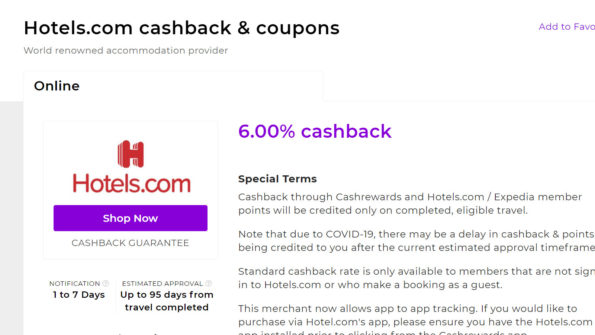Screenshot of a web page from Hotels.com showcasing cashback and coupon offers:

At the top of the page, a prominent header reads "Hotels.com Cashback and Coupons" followed by smaller, gray text stating "World-renowned accommodation provider" with the label "Online" beneath it. Below this, featured in purple text, is "6% Cashback" displayed as "6.00%". Directly underneath, in black text, the phrase "Special Terms" is displayed, detailing that cashback through cashback rewards and points from Hotels.com/Expedia will be credited only upon the completion of eligible travel.

A disclaimer about COVID-19 follows, along with extensive information regarding the standard cashback rate and app tracking details. 

On the left side of the web page, there is an image featuring the Hotels.com logo, adjacent to a purple "Shop Now" button. Below this button, the text "Cashback Guarantee" is visible. Another detail under this section indicates: "Notifications: 1 to 7 days, estimated approval up to 95 days from travel completion."

In the upper right-hand corner, a partially cut-off purple button labeled "Add to Favorites" is noticeable. The overall color scheme of the website comprises purple, black, white, and red, which corresponds to the colors in the hotels.com logo.